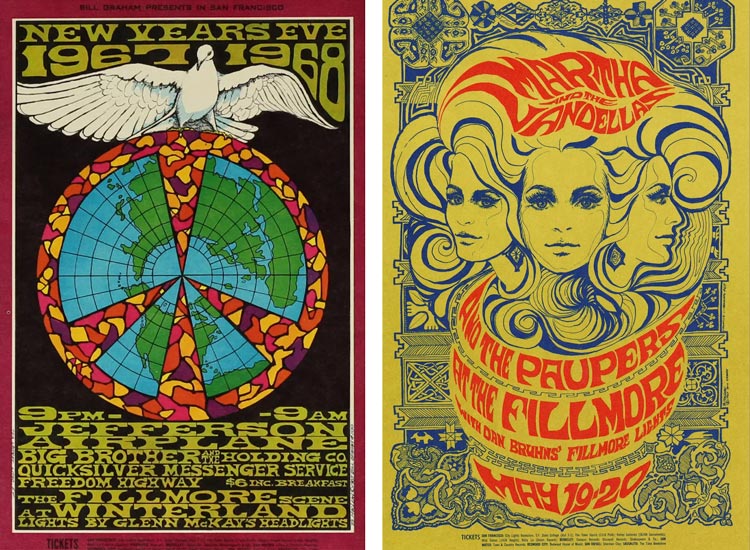The image showcases two adjacent psychedelic rock posters from the 1960s, designed in vibrant and flowing organic shapes. The poster on the left, set against a black background, announces a New Year's Eve concert for December 31, 1967, to January 1, 1968, featuring Jefferson Airplane, Big Brother and the Holding Company, Quicksilver Messenger Service, and Freedom Highway, held at the Fillmore at Winterland. The central artwork features a peace symbol encompassing a globe with green continents and blue oceans, encircled by a stained glass-like border of yellow, pink, orange, and purple. Above the globe, a white dove with outstretched wings is prominently displayed, with "New Year's Eve 1967-1968" inscribed in a brownish-green font over it. Beneath the main image, in green, psychedelic-style letters, are the concert details and band names.

The right-hand poster, predominantly in pale olive-green with intricate blue patterns, advertises a concert for Martha and the Vandellas, with The Poppers as the opening act, set for May 19th and 20th at the Fillmore, though the year is not specified. The poster features three women with surreal, flowing, psychedelic hair rendered in blue, and all the text, including the concert details, is in bold red and dark blue fonts, creating a striking visual contrast.